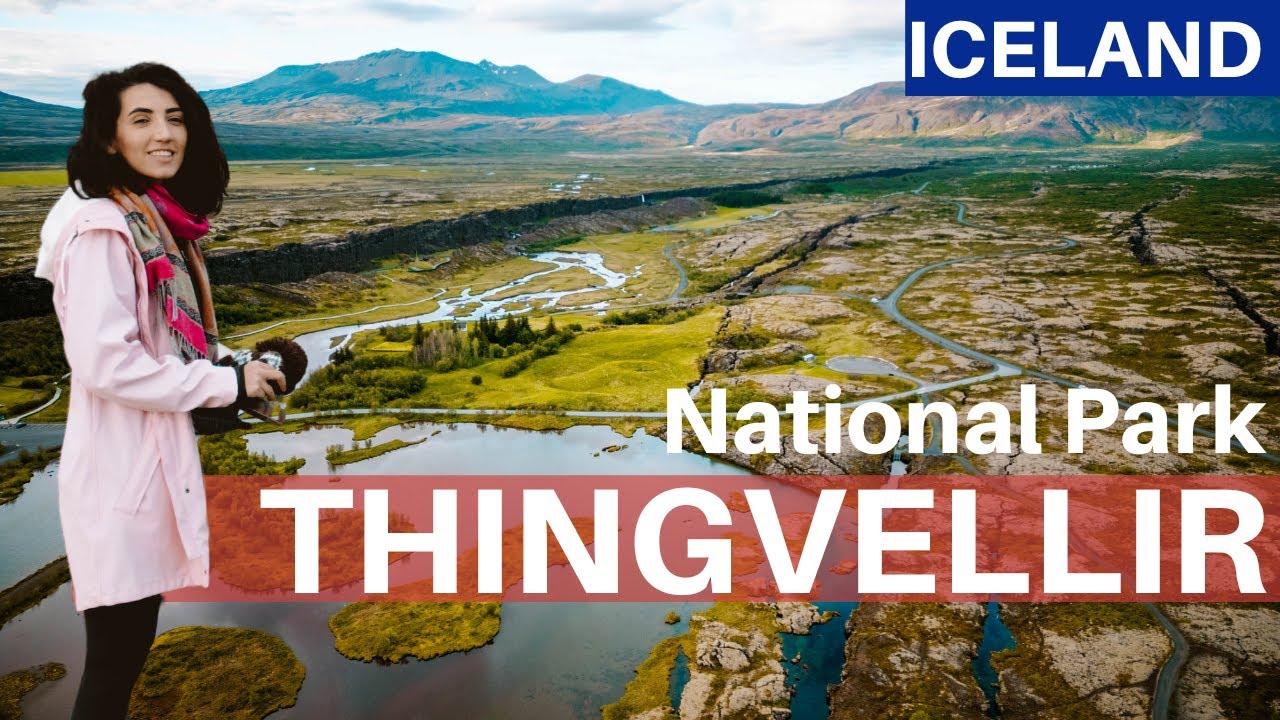This image, in a landscape layout, portrays a striking and expansive countryside scene in Iceland. The serene backdrop comprises green grassy plains, waterways, a large body of water with grassy islands in the lower left-hand corner, and a majestic mountain range under a blue sky with clouds. There is a blue text box in the upper right-hand corner with the word "ICELAND" in bold white letters. Below, in white text, it reads "National Park," and a red bar with white text displays "Thingvellir." On the left side of the image stands a woman with dark brown hair wearing a distinctive pink coat, a multicolored scarf in shades of red, tan, green, and blue, and black pants. She appears to be a travel guide, adding a human element to this breathtaking natural setting of Iceland's National Park Thingvellir.